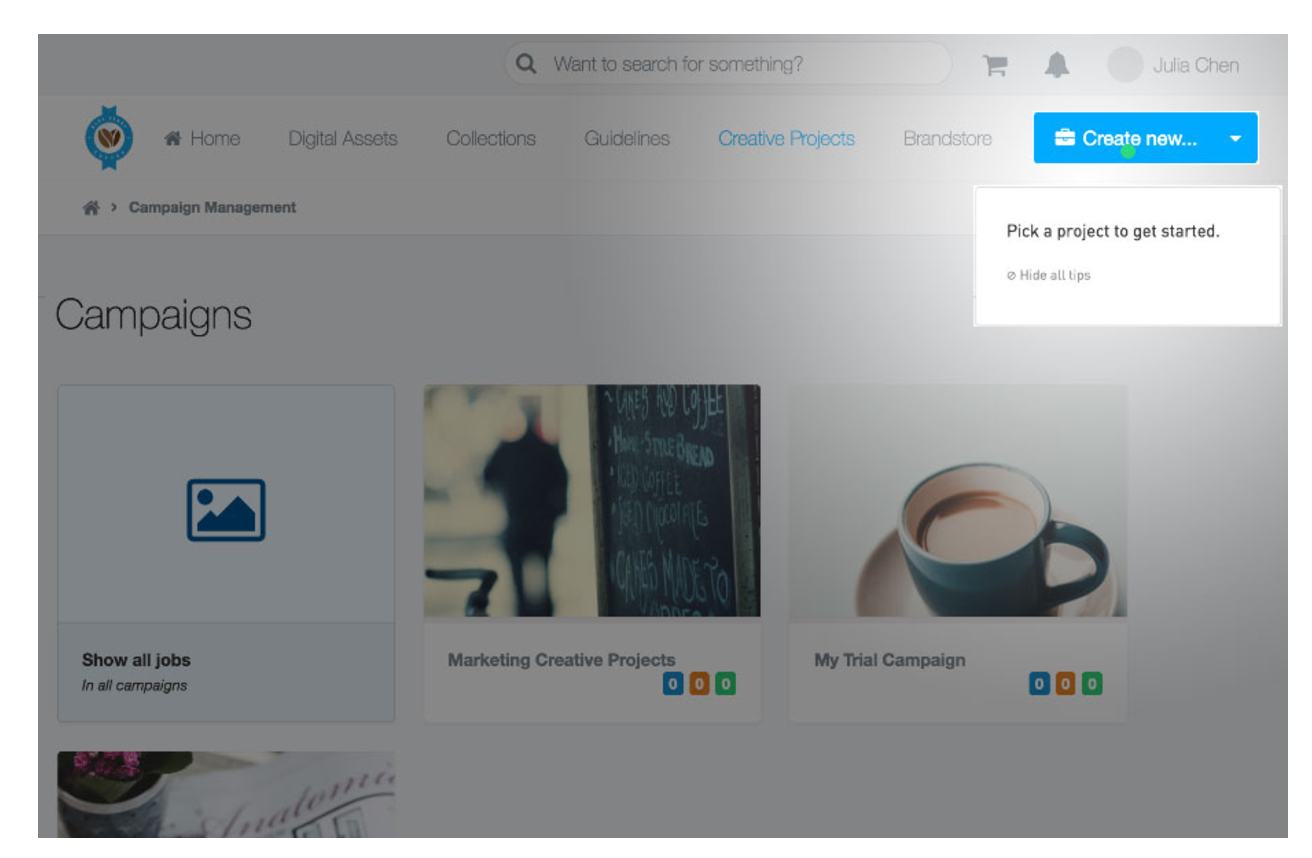This is a screenshot of a sales-oriented website, seemingly targeting new users. The main screen is dim, creating a spotlight effect on the top right-hand corner that highlights a button labeled "Create New," adorned with a green dot to draw attention. Below this button is a white text box containing the message "Pick a project to get started" in black text, followed by an option to "Hide all tips," indicating it's a tutorial or onboarding guide. 

The top left corner features the website's logo—a red heart with yellow veins extending from its sides. The bottom left corner has a section titled "Campaigns," showing various campaigns, possibly created by the user. One campaign, labeled "My Trial Campaign," is depicted with an icon of a coffee mug. Another, named "Marketing Creative Projects," shows an image of a person walking past a chalkboard.